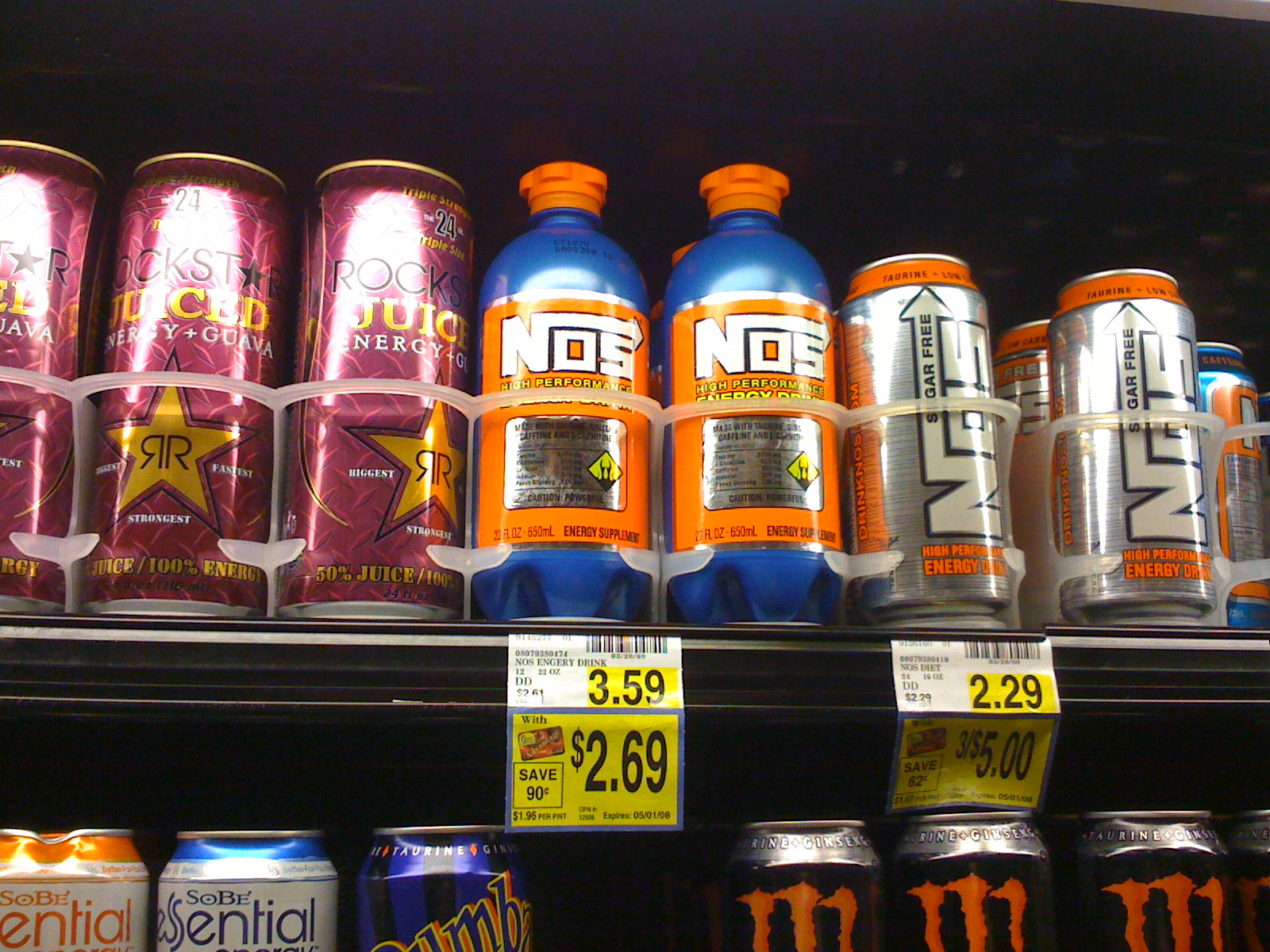In this image of a store shelf, we see a detailed and closely zoomed-in view of the upper half and the shelf above it, focusing primarily on a selection of beverages. At the bottom of the frame, the tops of several cans are visible. The can on the far left features an orange and gray indent, followed by a gray can with a blue cap. Next is a dark blue and black can, and adjacent to it are three Monster Energy Drink cans, each prominently displaying the iconic orange "M" logo. Above these cans are two price tags: the left tag reads "$2.69, save $0.90," while the right tag offers a deal of "three for $5."

On the top row, the three cans on the left are purple and labeled "Rockstar Juiced." To their right are two blue Nas bottles with orange labels and caps. Further to the right, there are gray Nas cans accented with orange tops and text. The background of the image is filled with black spaces, allowing the bold colors and branding of the drinks to stand out clearly.